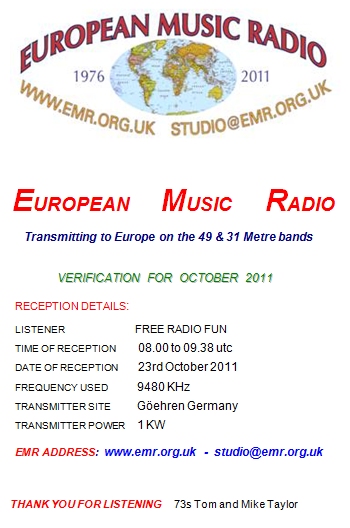The image features a white background primarily dedicated to details about European Music Radio. At the top is a colorful, oval-shaped globe with blue oceans and multi-colored continents. Surrounding the globe in a curved format are the words "European Music Radio" in prominent red text, alongside the timeline "1976-2011". Flanking the globe on either side are the URLs "www.emr.org.uk" and "studio@emr.org.uk."

Beneath the globe, again in red text, it states "European Music Radio transmitting to Europe on the 49 and 31-meter bands." Below this, in green text, it says "Verification for October 2011." The reception details follow in black text, reading: "Listener: Free Radio Fund," "Time of reception: 08:00-09:38 UTC," "Date of reception: 23 October 2011," "Frequency used: 9480 kHz," "Transmitter site: Göhren, Germany," and "Transmitter power: 1 kW."

Further down, in red text, it says "EMR address," followed by the URLs "www.emr.org.uk" and "studio@emr.org.uk" in blue. The image concludes with a thank you note in red text: "Thank you for listening," and in black text: "73S Tom and Mike Taylor."